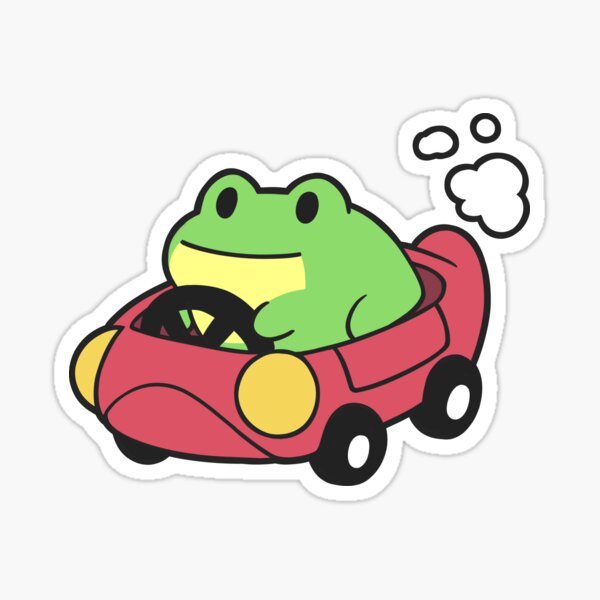This image is a charming, cartoon-like depiction of a green frog driving a small red car. The background is a solid, light gray with no text or border. The frog, which has black eyes and a yellow underside, appears content, wearing a gentle smile as it grips the black steering wheel with its left hand. The red car, outlined in black, features black tires with white rims and yellow headlights, one shown as a full circle and the other as a half circle. Thick black outlines accentuate the car's details, including the door and front end. Puffs of white smoke emerge from the car's exhaust, adding a playful touch to the animated scene. The overall style is whimsical and skillfully drawn, reminiscent of a children's comic or book illustration.